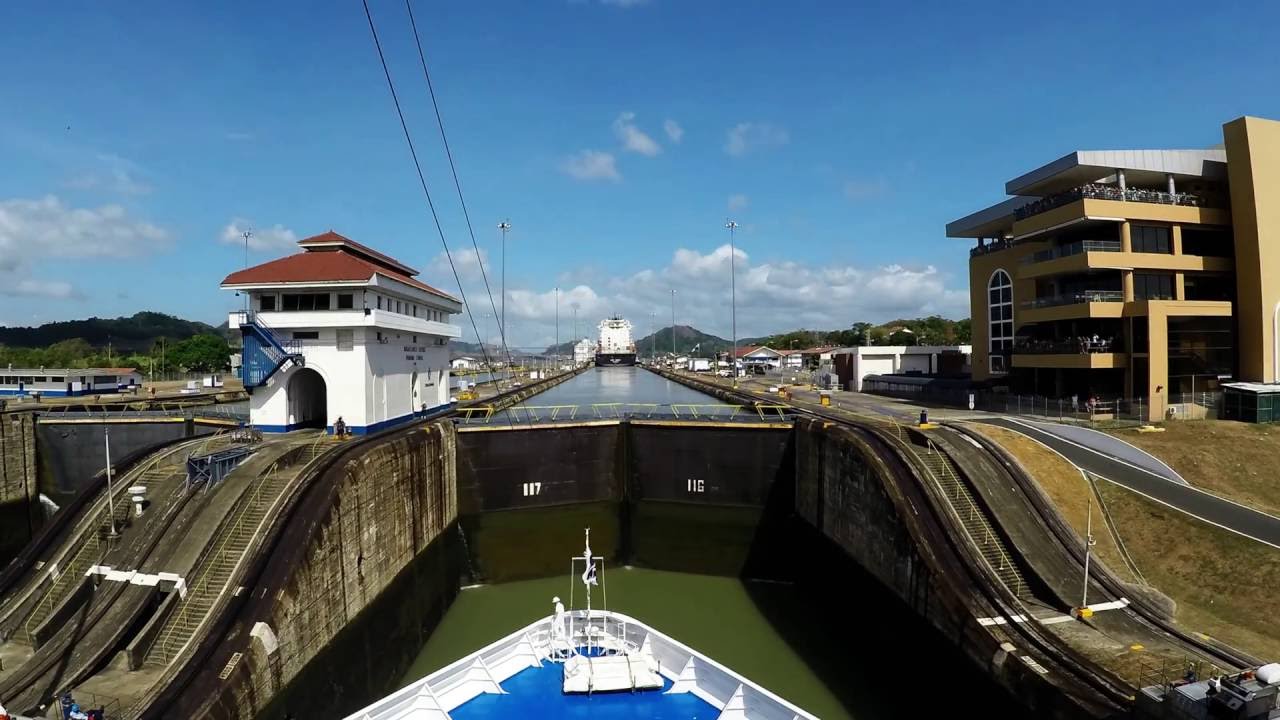This image is a color photograph capturing a ship navigating through a lock system at a dam, likely part of a significant canal such as the Panama Canal. The foreground prominently features the bow of a large ship, painted white with a blue deck. The ship is positioned within a massive concrete lock, with walls towering on either side and gates visible ahead, ready to regulate the water level.

On the left side of the image, there is a small white building, likely used by the personnel operating the lock system. Directly opposite, to the right side, stands a several-story yellow building with balconies. Metal tracks run alongside the ship, possibly used for maintenance or operational purposes.

The background reveals rolling green hills and scattered trees, with another ship visible further down the canal, suggesting ongoing traffic through this waterway. Overhead, a blue sky dotted with clouds stretches across the upper half of the image, with poles and wires—likely for communication or power—crossing the scene. The entire composition underscores the engineering marvel of the lock system and its integration with the surrounding landscape.